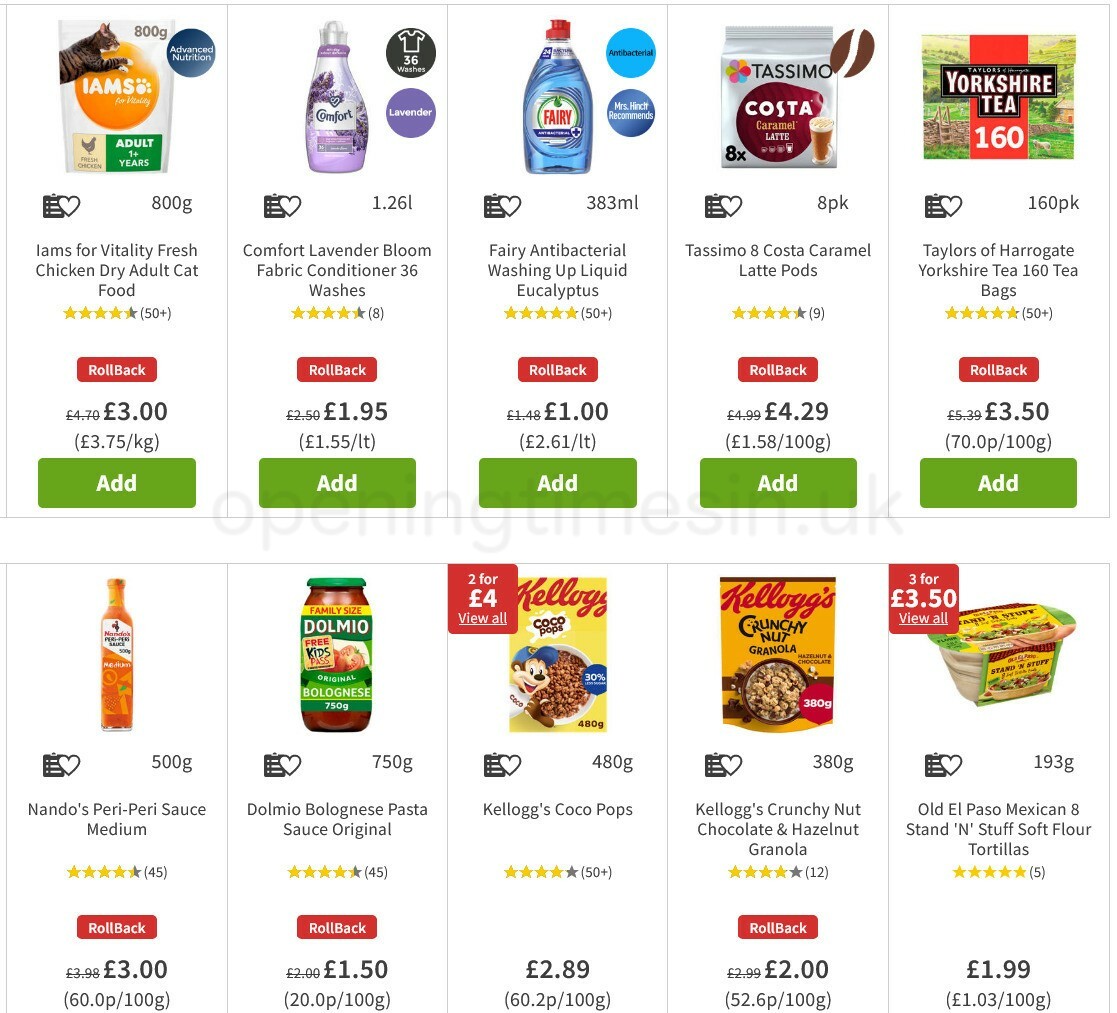In the image, there is a neatly organized grid displaying various marketplace food products and household items. Some of the products featured include Iams cat food, lavender-scented fabric conditioner, antibacterial liquid soap, dish soap, caramel latte pods designed for a Keurig or similar coffee maker, Yorkshire tea bags, peri-peri sauce, pasta sauce, Coco Pops cereal, Kellogg's Crunchy Nut cereal, chocolate and hazelnut granola, and Old El Paso Mexican flour tortillas.

Each item is clearly marked with its price in British pounds (£), and every product boasts a review rating of at least 4 out of 5 stars. Among the array, the dish soap, priced at £1, stands out with the highest ratings. Beneath each product is a prominent green "Add" button for easy purchase. The image snapshot provides a comprehensive view of various well-reviewed items available in this online marketplace.